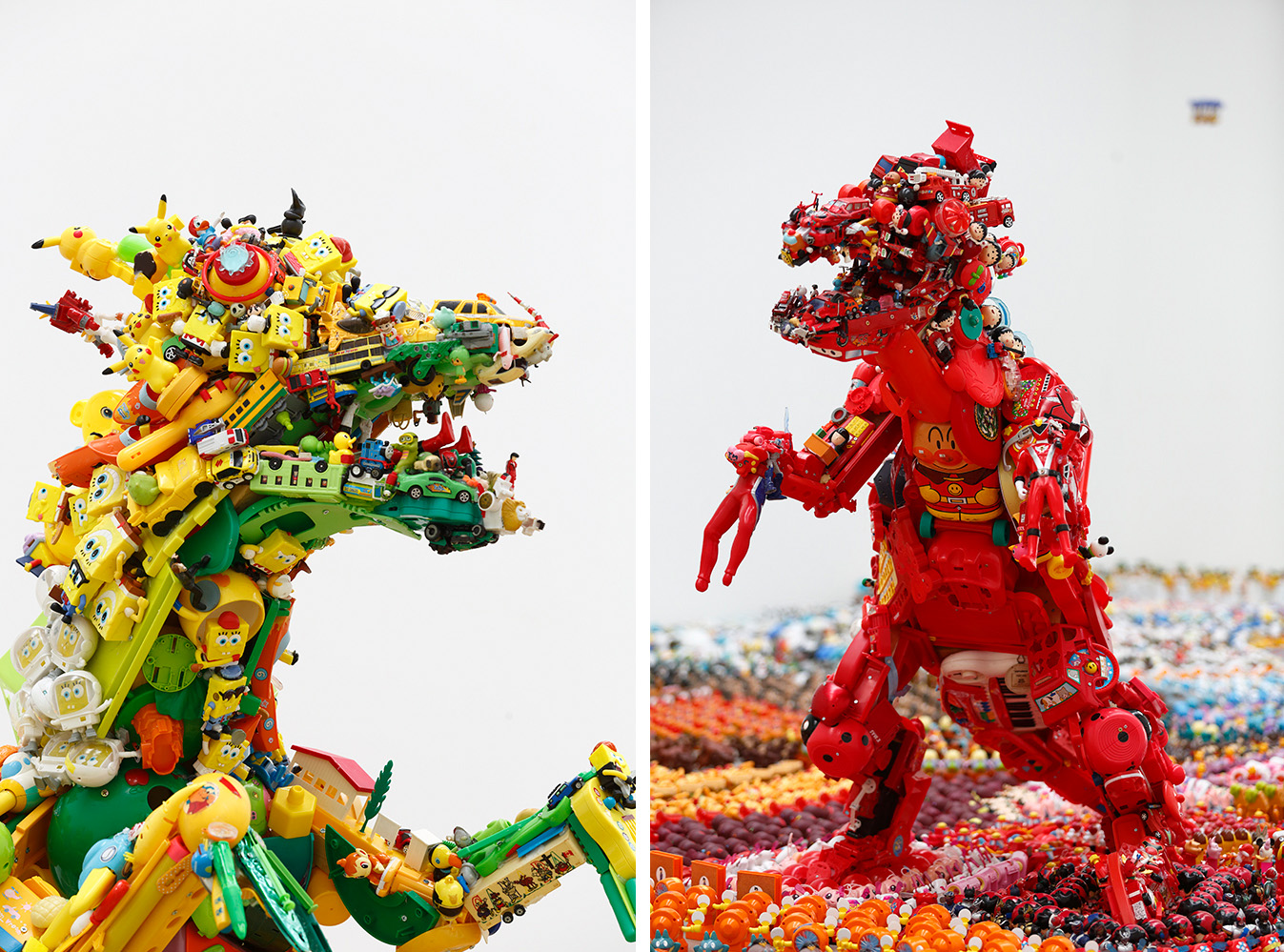In this composite image, there are two separate digital images displayed side by side, each featuring a dinosaur sculpture made up of smaller toys. The left sculpture is predominantly green and yellow, composed of a variety of toys including green and yellow cars, SpongeBob characters, and Pikachu figures. It resembles the upper body of a dinosaur with its head and open mouth prominently visible. The right sculpture, on the other hand, is primarily red and slightly orange, containing toys such as fire trucks, red action figures like a Power Ranger, and various other red and blue toys. This dinosaur sculpture stands on a base made of additional toys, and its full body is visible. Both sculptures are set against a white or light blue background, presenting a colorful and intricate collage of recognizable small toys.